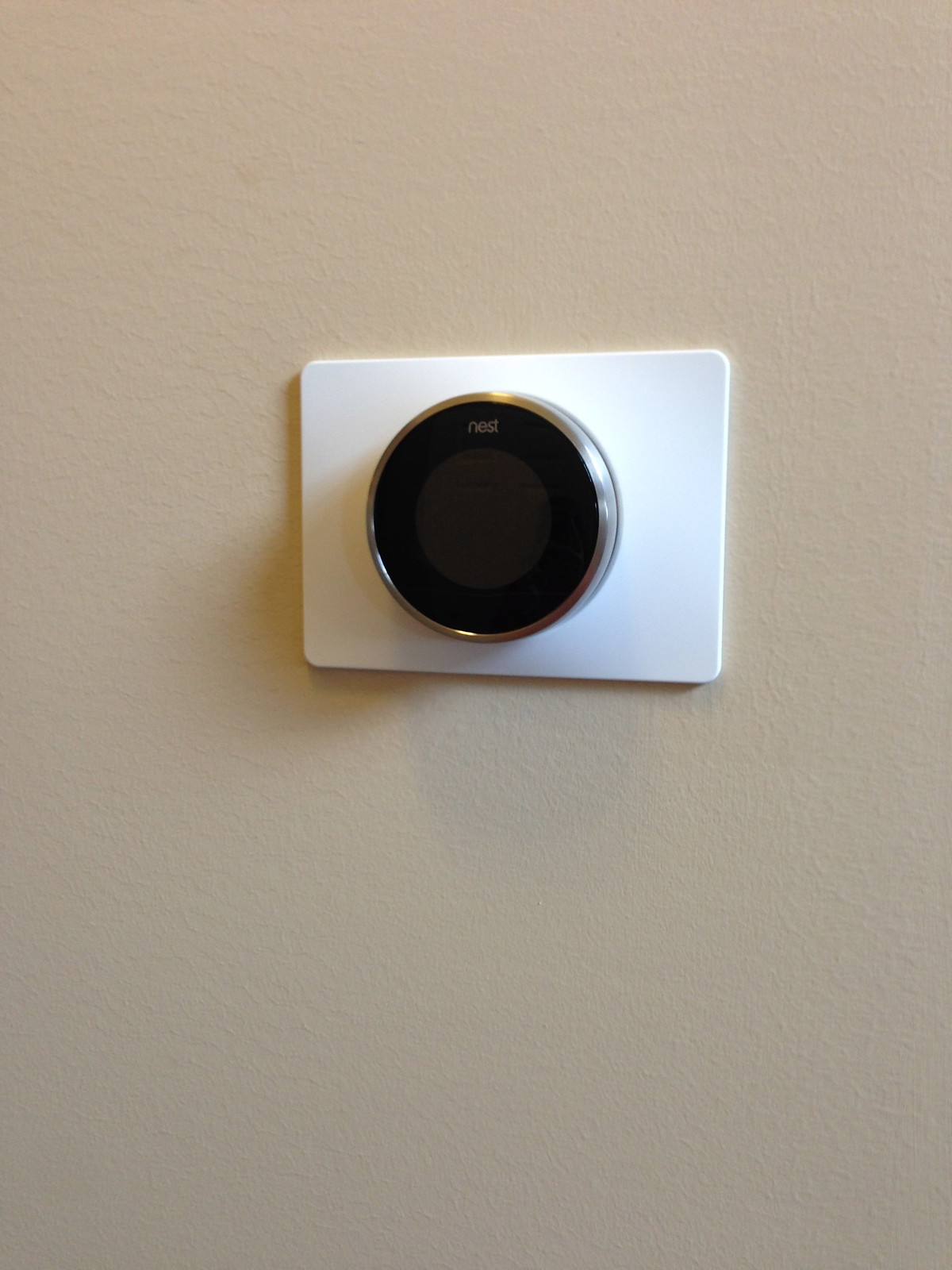The image features a tan-beige wall with an orange peel texture, giving it a subtly rough appearance. Mounted almost perfectly in the center of the image is a metallic or iridescent white square panel that closely adheres to the wall. The focal point of this panel is a sophisticated Nest smart thermostat. 

The thermostat, seemingly turned off, is composed of several distinctive elements. At its core is a silver ring that serves as a knob. Encircling this silver knob is an outer black ring. Nested within the center of the silver ring is a transparent black circular touchscreen. At the top of this black outer ring, the brand name "nest" is displayed in lowercase white letters.

The device is illuminated by a light source positioned at the top-right of the image, casting a diagonal shadow to the left. This lighting creates multiple flashpoints on the thermostat's silver ring, highlighting its polished finish with gleams at the top, sides, and bottom. The sleek design of the thermostat ensures the white panel scarcely protrudes from the wall, maintaining an almost flush appearance.